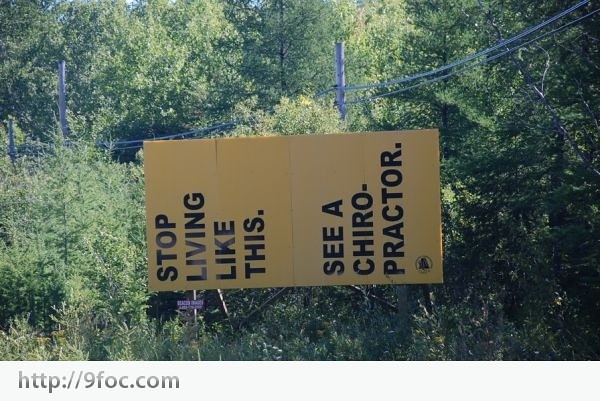The photograph, taken outdoors in landscape orientation, features a prominent yellow placard with black writing that is incorrectly oriented horizontally. When correctly rotated 90 degrees clockwise, the sign displays two messages in stacked squares separated by a horizontal line. The top square, in bold capital letters and left-justified, reads, "STOP LIVING LIKE THIS." The bottom square contains the text "CA CHIRO- PRACTA," split across multiple lines. Below the sign, there's a light cream-gray strip with the URL "http://9foc.com." The background reveals an untamed wilderness with dense green foliage, trees, and bushes, indicating a poorly maintained area. Additionally, two telegraph poles are visible—one on the right and one in the background to the left—connected by wires crossing the upper section of the image.